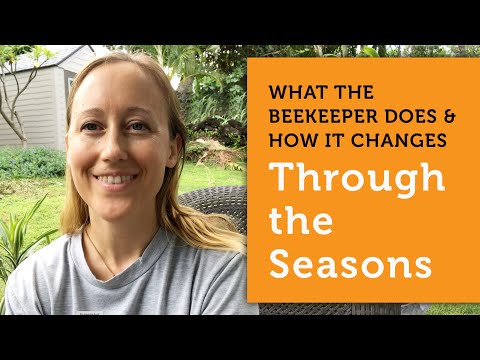This image seems to be a screen capture from a commercial or an advertisement, possibly for a magazine or even a YouTube thumbnail. In the background, we see a cheerful Caucasian woman seated in a wicker lawn chair, enjoying her backyard. She is wearing a light gray t-shirt and has long, fine blonde hair with minimal makeup. The setting features lush greenery, including bushes, trees, and well-maintained grass, along with a small shed. To the right of the image, there is an orange box containing text that appears to be professionally added via graphic design software. The text, featuring a drop shadow effect, reads "what the beekeeper does and how it changes through the seasons," with the phrase "the seasons" in white font and the rest in black. The image is framed by black borders at the top and bottom, giving it a constrained aspect ratio.